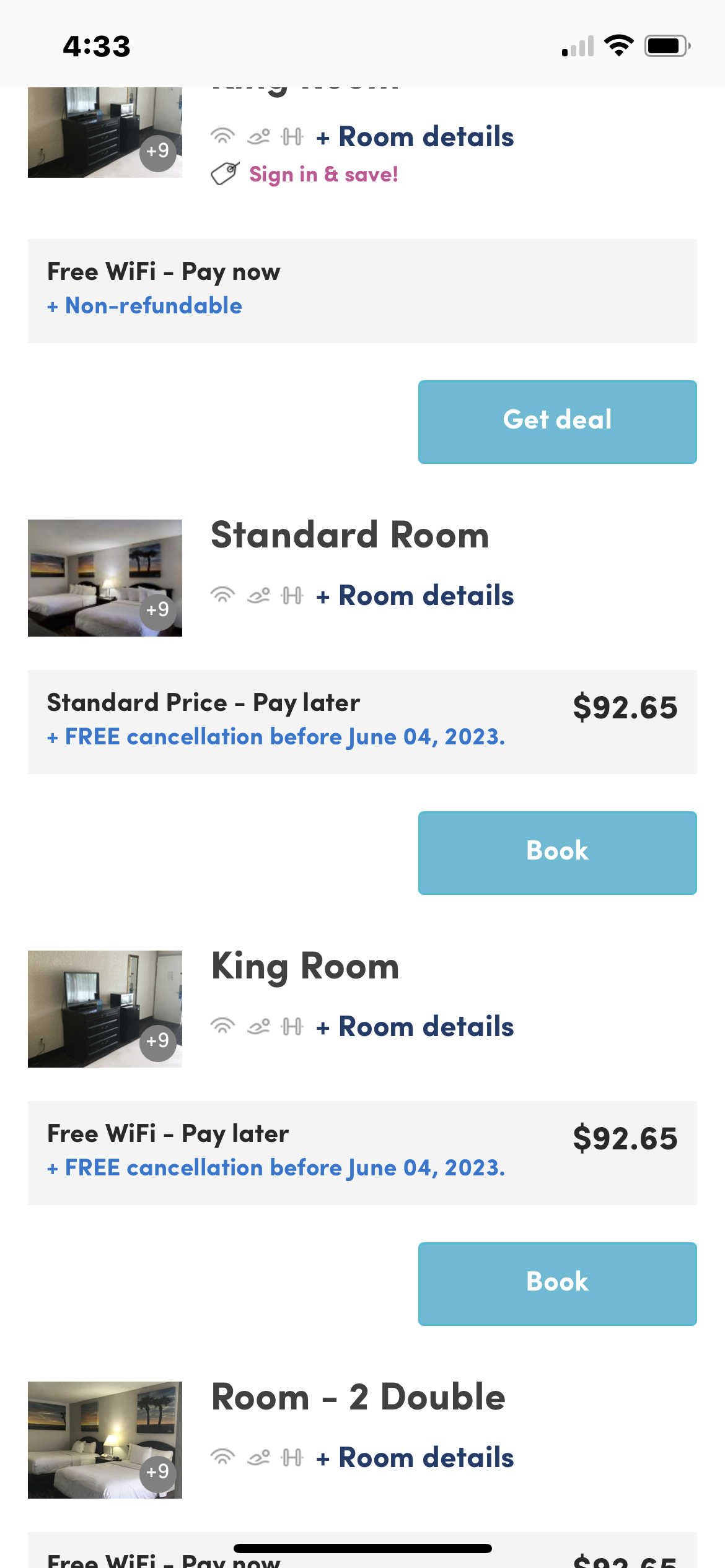This is an image that appears to be a screenshot taken from a phone. The upper part of the screenshot features a light gray banner displaying the number "4:33" in bold in the left-hand corner. To the right, there is a signal bar showing one filled bar out of four, followed by a fully filled Wi-Fi signal icon, and then a fully charged battery icon.

Below this banner, an image is partially visible, hinting at a possible room with what looks like parts of a bed and a dresser. To the right of the image, there is a gray circle with the text "+9" inside it. Adjacent to this, "Room Details" is written, and next to it, there is a maroon-colored text saying "Sign in and save", accompanied by a coupon icon on the left.

Underneath this section is a light aqua blue button labeled "Great Deal". Near the center of the image, the text "Standard Room" appears, with a small image of two beds featuring a "+9" icon to its left. Again, "Room Details" is written to the right. Below this, in a gray banner area, it says "Standard price paid later: $92.65". Another text with similar information follows, ending with a "Book" button at the bottom.

Further down, the "King Room" type is displayed in a similar format with another "Book" button and a corresponding price. Lastly, there is a section labeled "Room to Double," but the accompanying details and price are cut off.